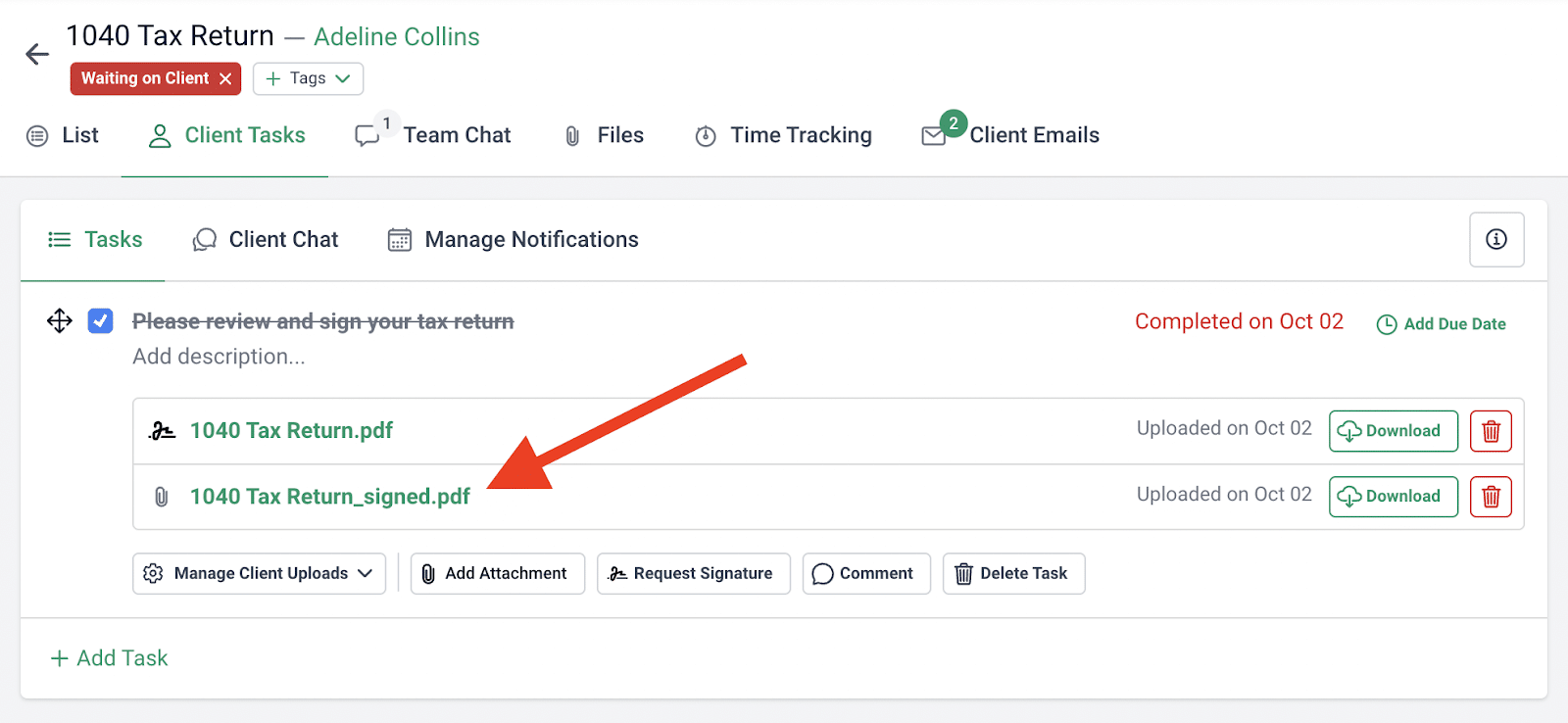The image is a horizontal rectangle with a white background and various sections of text and icons. At the top, it features a bold black text stating "1040 Tax Return—" followed by green text reading "Adeline Collins," which appears to be fully capitalized as "CO LLINS." 

Below this is a horizontal red rectangle containing the white text "Waiting on Client" with a small white "X" next to it. Between this red area and the aforementioned text is a small left-facing arrow. Adjacent to the red area is a white rectangle labeled "Tags" in black font, preceded by a green plus symbol and followed by a green downward arrow.

The menu on the left side features several items, each prefixed with an icon:
1. "List Client Tasks" in green.
2. "Team Chat" with a thought bubble icon and a tiny "1" next to it.
3. "Files."
4. "Time Tracking."
5. "Client Emails" with an envelope icon that has a green circle containing the number "2" in white font.

Further down, there is a green icon with three horizontal lines and the text "Tasks" with a capital 'T.' Below this, in black text, are "Client Chat" and "Manage Notifications."

In the main content area, a blue square with a white check mark houses the text "Please review and sign your tax return," which is crossed out. Below this text is the option "Add Description" in normal font, followed by two documents:
1. "1040taxreturn.pdf" in green.
2. "1040taxreturn_sign.pdf" in green, pointed to by a bold red arrow indicating it is the signed copy.

To the right of "Please review and sign your tax return," in red text, it states "Completed on October 02." Nearby, in green text, is the option "Add Due Date."

Next to the first document, it says "Uploaded on October 02" in green text. Below both documents are two options in white text within green and red boxes:
1. A green box that says "Download" with a download icon.
2. A red vertical box with a white trash can icon.

The bottom section contains black text options:
1. "Manage Client Uploads."
2. "Add Attachment."
3. "Request Signature."
4. "Comment."
5. "Delete Task."

In the lower left-hand corner, a green plus sign followed by "Add Task" is visible.